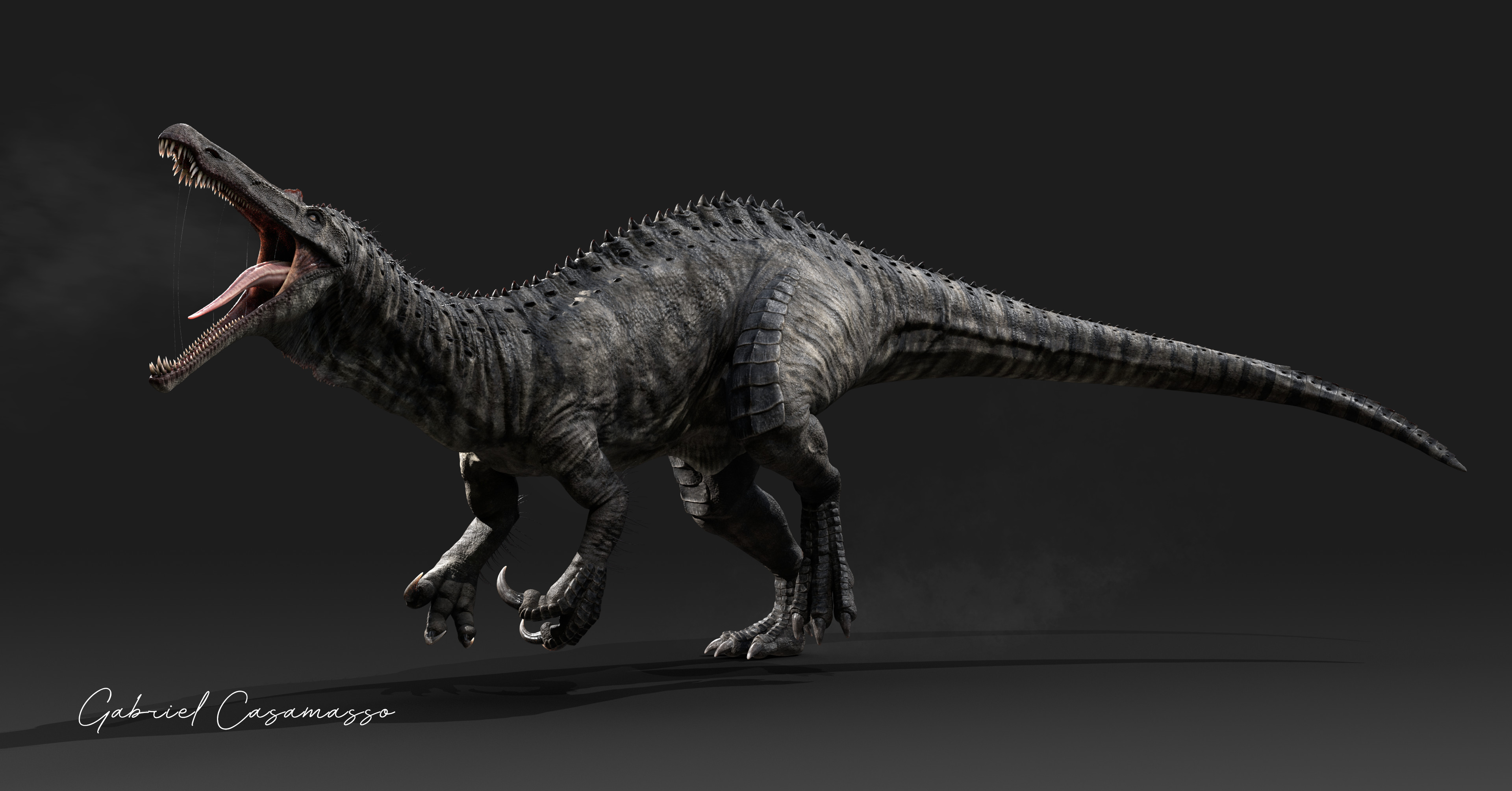The digital image showcases a highly detailed, realistic 3D model of a dinosaur against a black background with light gray fog swirling around it. The ground is also black, casting a distinct shadow of the dinosaur. The creature resembles a Spinosaurus, characterized by a long, slender alligator-like snout lined with numerous tiny teeth and a sharp, pointy tongue hanging out, giving the impression that it's roaring. Its arms are noticeably longer than those of a T-Rex and are equipped with large, bladed claws. The dinosaur's body is dark-colored, with intricate details depicting scales and wrinkles, and it possesses a rugged, saw-blade-like ridge running down its back. The muscular hind legs support a very long, pointed tail. In the bottom left corner of the image, there is a signature: Gabriel Kagamasa.